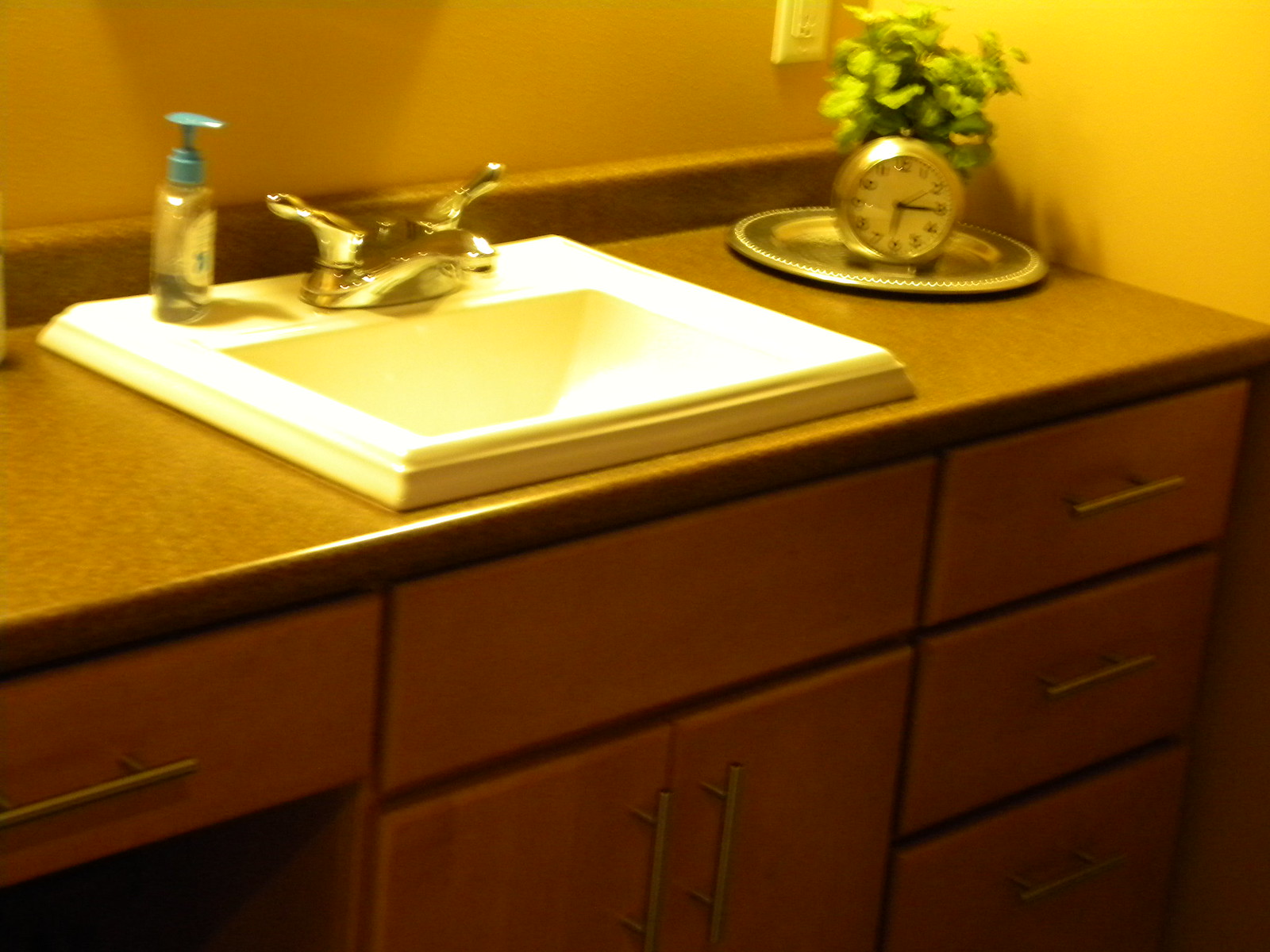The image captures a detailed view of a bathroom sink from a top-front angle. The walls surrounding the sink are painted a soft yellow hue, providing a warm ambiance. The countertop features a granite finish, with lighting that casts a subtle brownish tint. In the top right corner of the countertop, there is a small round tray that holds a metallic analog alarm clock with a white face, set to 6:15. Behind the clock, a small plant is sprouting, adding a touch of greenery to the scene.

The sink itself is white and square-shaped, accompanied by a metallic faucet and handles. A transparent bottle of hand soap with a teal-colored dispenser is placed next to the faucet. Below the sink, the cabinetry is a rich brown adorned with metal handles, including the visible drawers that share the same design. The overall composition highlights both functionality and aesthetic detail.